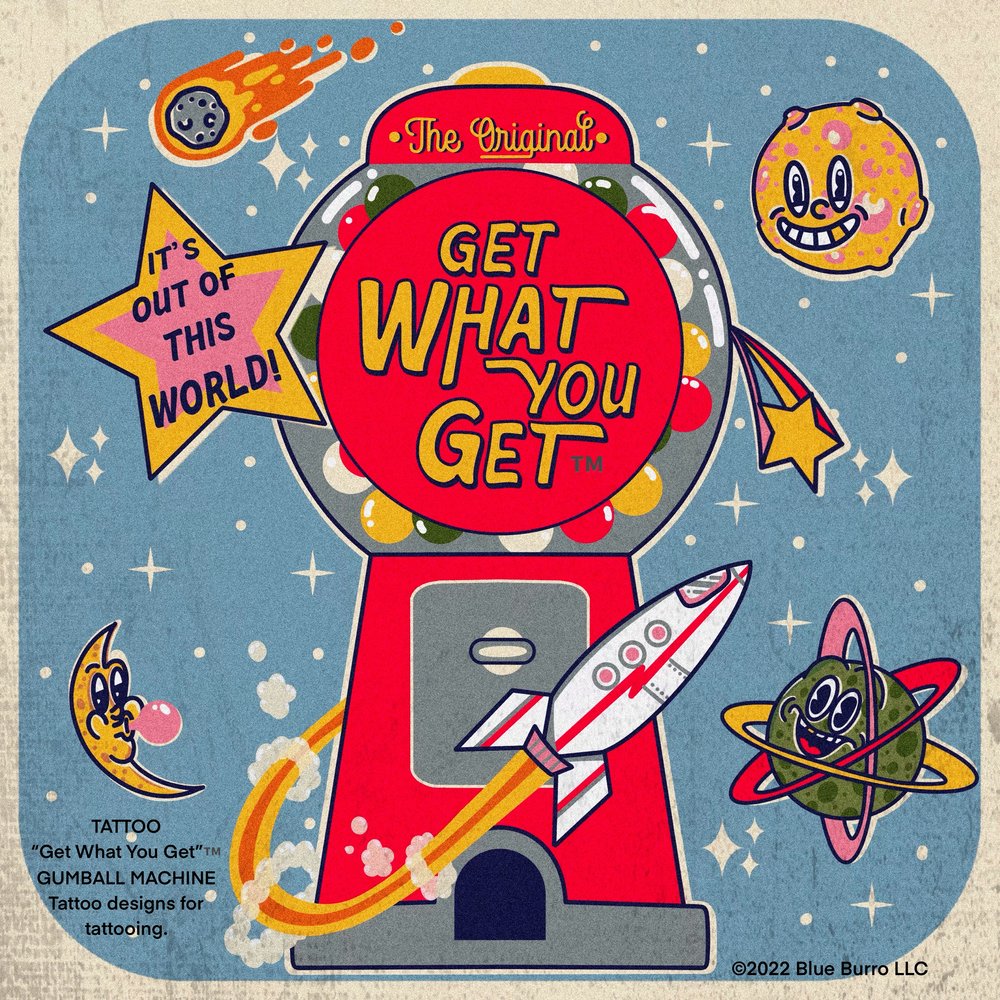This vibrant and colorful advertisement, designed with a retro space theme, features a detailed drawing of a classic red gumball machine against a cream-colored background. The main headline in orange script reading "The Original" and "Get What You Get" circles around the gumball machine. At the bottom left, a label states, "Tattoo - Get What You Get Gumball Machine Tattoo Designs for Tattooing," emphasizing that the machine dispenses random tattoo designs as its prizes. A playful, mid-century modern style is evident with various space motifs, including a smiling Saturn in the top right corner, a cheerful moon blowing a pink bubble, a lively rocket blasting off from the bottom, and a dynamic meteor in the top left. To the left of the machine, a pink star with a blue-font message outlined by a yellow star says, "It's Out of This World." Completing the whimsical scene, an atom with colored rings and light blue and white stars against the cream backdrop enhance the design. The lower right corner notes the copyright as 2022 Blueboro LLC.